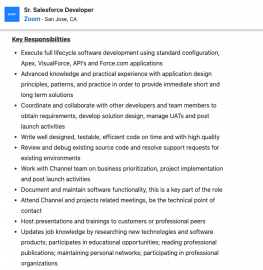Caption:

A screenshot of a web page detailing the qualifications and responsibilities for the role of "Senior Salesforce Developer" based in San Jose, California. The top section prominently displays the job title. To the left side of the page, a blue square icon is featured, accompanied by the caption "Key Responsibilities" below it. The page outlines various key responsibilities in black text, each preceding a detailed bullet point explanation. The first listed responsibility is to “execute full lifecycle software development" using tools and technologies like standard configuration, Apex, Visualforce, APIs, and Force.com applications. Additional responsibilities include documenting and maintaining software, as well as hosting presentations and training sessions for customers or professional peers. The web page has a minimalist design with a white background and a light gray divider separating the developer's name from the detailed key responsibilities, underscoring the straightforward and professional layout.